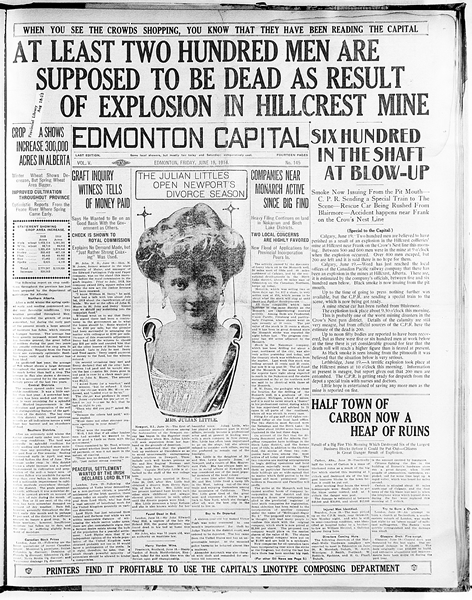This is a vertically aligned, black-and-white photograph of an old newspaper clipping from the Edmonton Capital, dated Friday, June 18, 1918. Dominating the page in bold, all-caps black print, the headline declares, "AT LEAST 200 MEN ARE SUPPOSED TO BE DEAD AS RESULT OF EXPLOSION IN HILLCREST MINE." Another stark heading on the far right states, "600 IN THE SHAFT AT BLOW UP." Below the main headline, smaller text is too fine to read, but several article headings provide more stories: on the left, "Crop Shows Increased 300,000 Acres in Alberta"; lower and to the right of it, "Graft Inquiry Witness Tells of Money Paid"; in the center, accompanied by a portrait of a woman with an elaborate hairstyle, "The Julian Littles Open Newport's Divorce Season"; next to it, "Companies Near Monarch Active Since Big Find"; and on the lower right, "Half Town of Carbon Now A Heap of Ruins." The bottom of the page reads, "Printers Find It Profitable To Use The Capital's Linotype Composing Department."